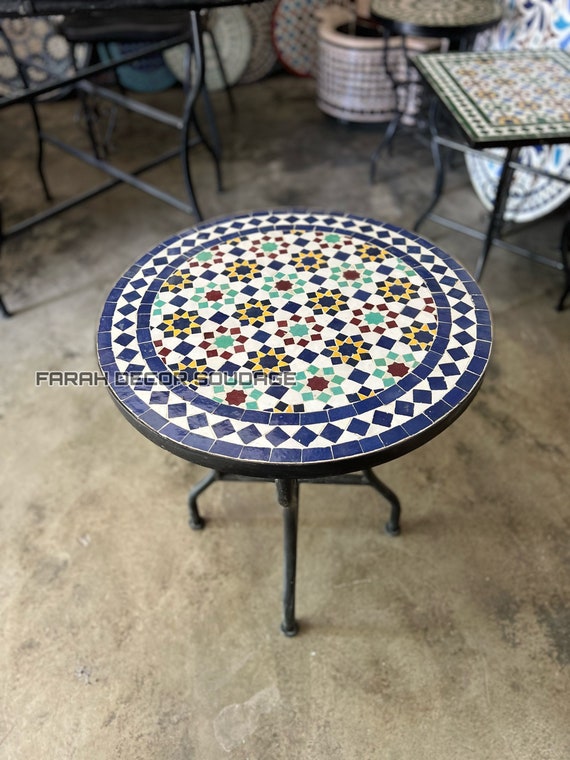This image captures a beautifully intricate round patio table adorned with a vibrant mosaic tile design. The tabletop features a strikingly detailed pattern, with the outer edge lined with blue tiles forming triangles and rectangles. Within this border, the design transitions into a mesmerizing array of blue diamonds set against a white background, interspersed with more blue rectangles. The centerpiece of the table showcases an elaborate floral motif, comprising rows of alternating blue, yellow, green, and red flower designs with various inserts, creating a captivating and colorful mosaic. The table stands on a sturdy black iron base with four legs, placed on a tan and black concrete floor. In the blurred background, additional tables and furniture suggest that the setting might be a furniture store. The image is overlaid with the text "Ferra Decor Sojourner," indicating that the table is likely part of a sale or display. The photo is taken from an overhead perspective, emphasizing the intricate and vivid details of the mosaic design.